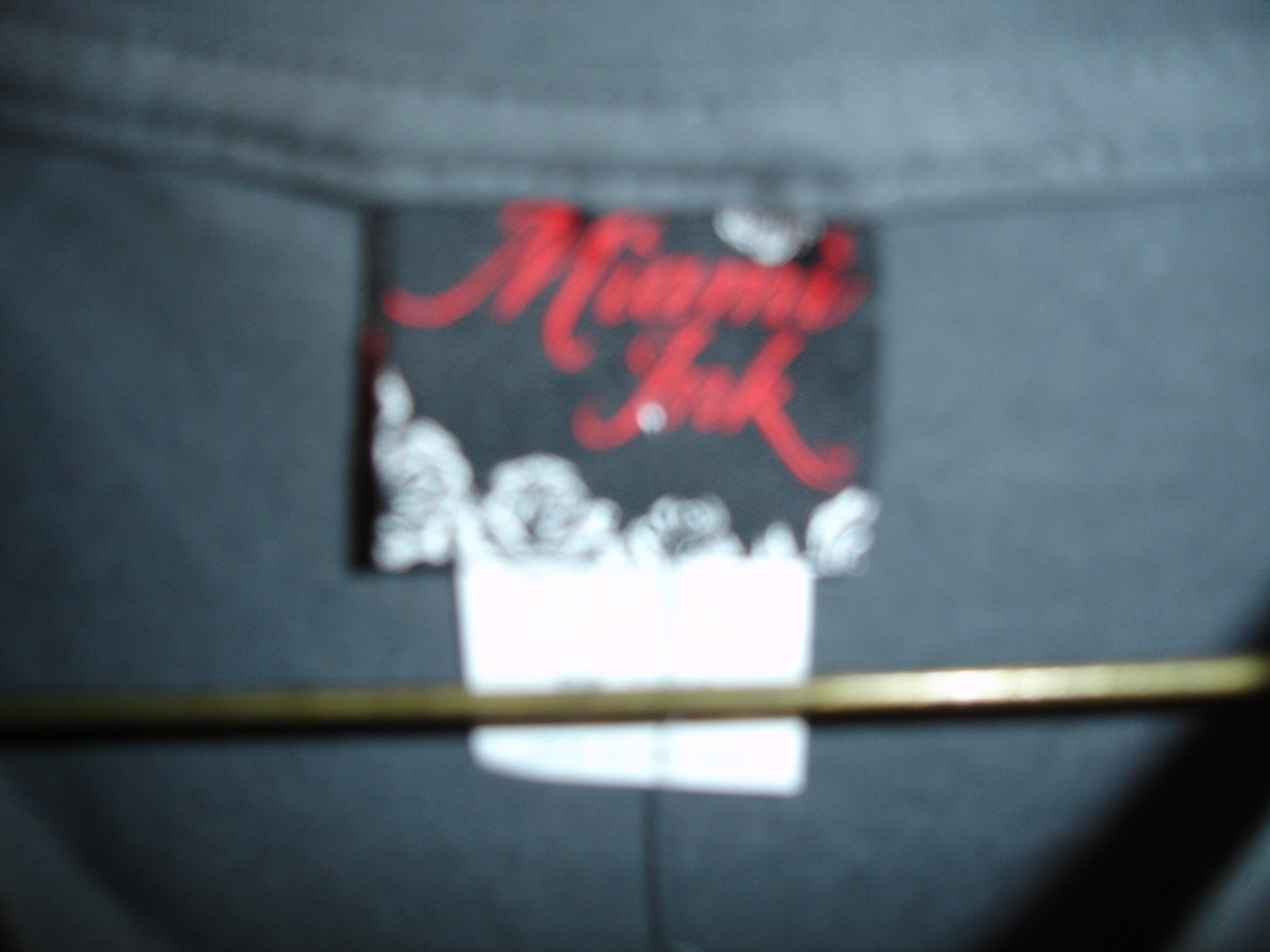In this close-up image, the focal point is a tag affixed to the inside of a dark gray shirt. Due to the proximity of the shot, the image is somewhat blurry, though certain details remain discernible. The stitching of the shirt is visible above the tag, forming two horizontal lines that extend across the frame. The tag itself is black, roughly measuring four inches in height and five inches in width. 

Prominently displayed in red text on the tag appears to be the word "Miami," spelled out as "M-I," followed by what may be an "A" or an "O," and then another "M-I." Below this, in red cursive script, the word "ink" can be faintly made out. Adding to the detail, a delicate white design embellishes the bottom of the black tag, though its exact pattern is indistinct.

Beneath this primary tag, a smaller white square tag is visible. Additionally, there is a narrow, gold or brass-colored strip, about an inch in height, stretching horizontally from the left edge to the right edge of the image. The combination of these elements suggests a branded garment, possibly from a collection labeled "Miami Ink."